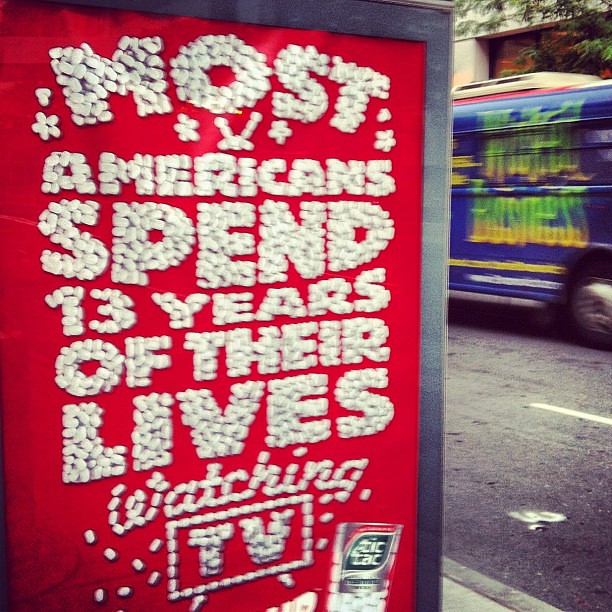The image depicts a street-level billboard advertisement for Tic Tacs, commonly seen in urban settings. The advertisement features a striking red background with a clever design: the message "Most Americans spend 13 years of their lives watching TV" is intricately spelled out using Tic Tacs. In the background, to the right, there is a partially blurry bus driving to the left, indicating the photo was taken in motion. Surrounding the bus are a few trees, adding a touch of greenery to the cityscape. The entire image has a slight blur, suggesting a candid, dynamic city environment.